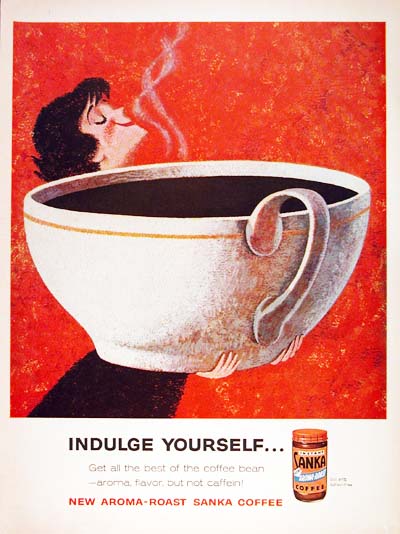This advertisement for New Aroma Rosanka Coffee is visually striking, featuring an artistic rendering of a woman savoring the aroma of a steaming, oversized coffee cup. The upper three quarters of the image are dominated by a rusty red background with a sketched, almost surreal depiction of the woman with black hair, dressed in black, holding a giant white cup with gold trim, which is filled with black coffee. Her face is tilted upward, inhaling the steam that whisks upwards from the cup, capturing the rich, enticing aroma. Below this image, on a white backdrop, the text reads, "Indulge Yourself. Get all the best out of the coffee bean: aroma, flavor, but not caffeine." Further down, in orange text, it introduces "New Aroma Rosanka Coffee." There is also a small illustration of the Sanka coffee labeling, which is distinctively orange, providing a complete visual and descriptive experience of indulging in a caffeine-free coffee rich in aroma and flavor.